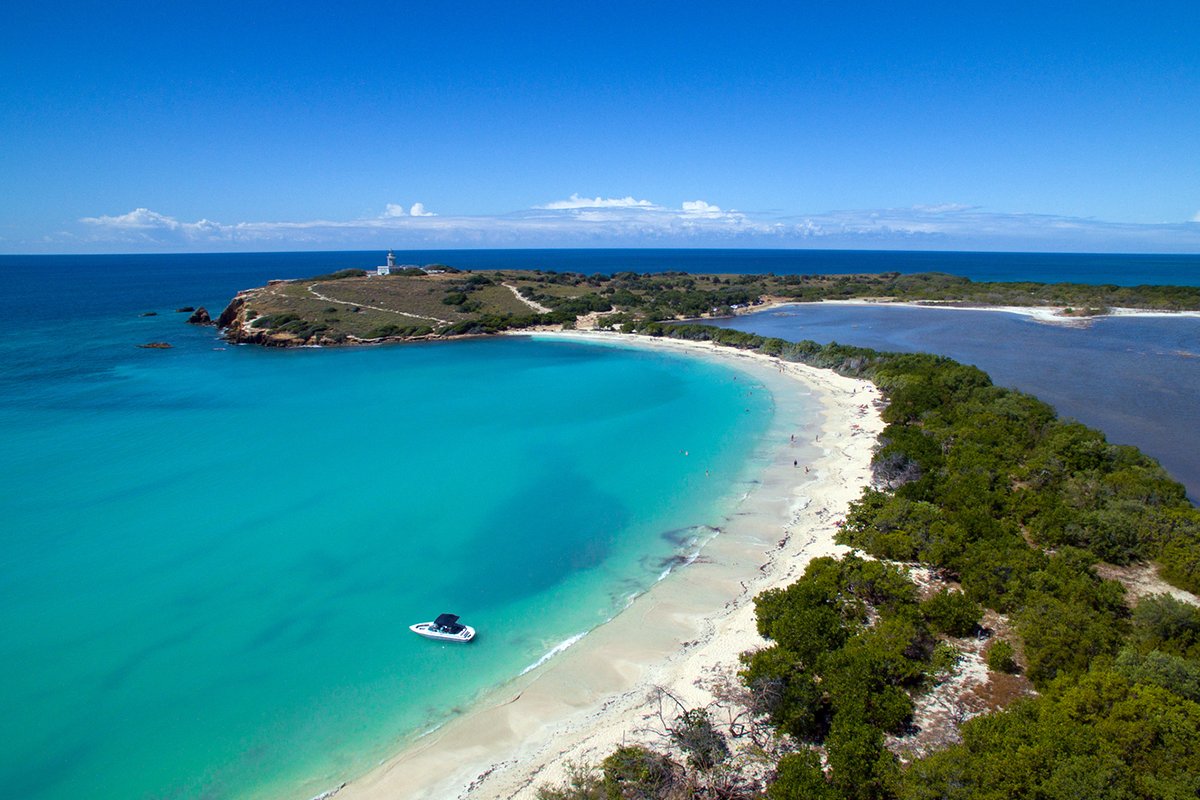This professional aerial photograph captures an exquisite coastal scene featuring a long, winding stretch of land bordered by crystal-clear, aquamarine blue waters. The coastline curves gently, almost forming a mini island with water on either side. The pristine white sandy beach is dotted with green trees and lush shrubbery, creating a picturesque natural setting. Anchored about 20 feet from the shore, a small white boat with a blue canvas top rests where the sand meets the sparkling water. The serene scene is accented by a distant lighthouse perched on a hill to the left, standing alongside a gray-roofed house and additional buildings at its base. The sky above is a vivid blue, punctuated by a few fluffy white clouds on the horizon. The absence of people in one part of the beach adds to the untouched paradise feel, while a few individuals in another section lend a sense of scale and serenity. The clean composition, vivid colors, and excellent lighting make this image magazine-worthy, perfect for a travel brochure.